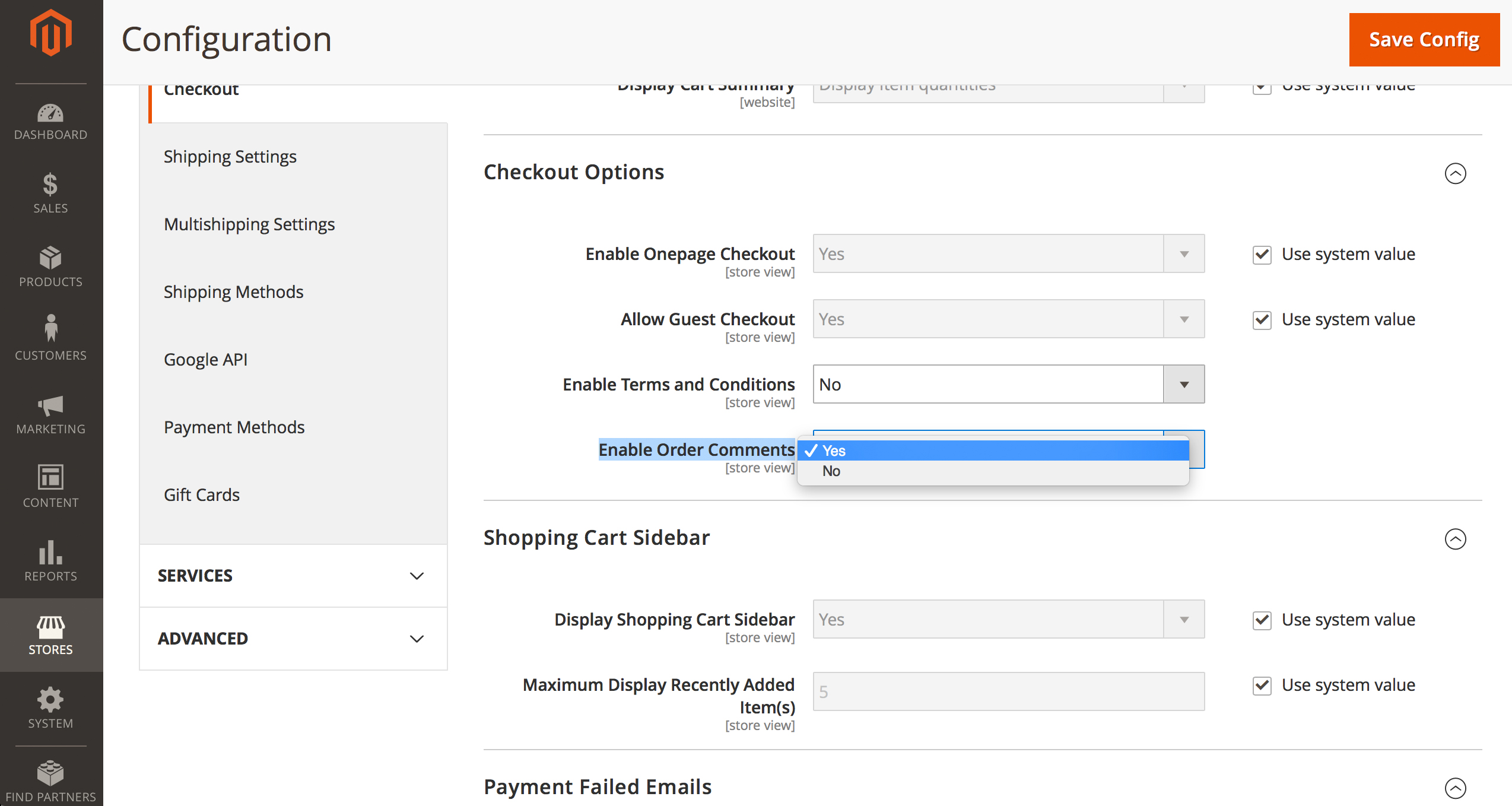The image depicts a configuration menu from an unidentified software platform, likely related to e-commerce management, as indicated by the various settings and options. In the upper left corner, there's a distinctive logo resembling a letter "U" with portions of an octagon surrounding it. Below the logo is a vertical navigation column featuring several icons, each representing different sections: a dashboard with a small meter icon, sales denoted by a money sign, products symbolized by a box, customers marked with a person icon, marketing indicated by a bullhorn, content tagged with a clip icon, reports shown with a graph, stores represented by a storefront, system settings marked by a cogwheel, and a final option for finding partners.

The highlighted section is "Stores," which is grayed out to indicate that it is currently selected. The main content area displays various store settings, including:

- **Checkout Options**
  - Enable one-page checkout: Yes
  - Allow guest checkout: Yes
  - Enable terms and conditions: No
  - Enable order comments: Yes

- **Shopping Cart Sidebar**
  - Disable shopping cart sidebar: Yes
  - Display recently added items: 5

Each of these options includes a checkbox to "use system value," which is currently selected. Additional sections include "Shipping Settings," "Multi-Shipping Settings," "Shipping Methods," "Google API," "Payment Methods," "Gift Cards," "Services," and "Advanced," all potentially expandable via dropdown arrows that are not currently activated. Lastly, there's a partially visible section for "Payment Failed Emails."

The overall interface features a clean white background with subtle gray highlights, and the selected column has a dark black background with an orange accent matching the logo.